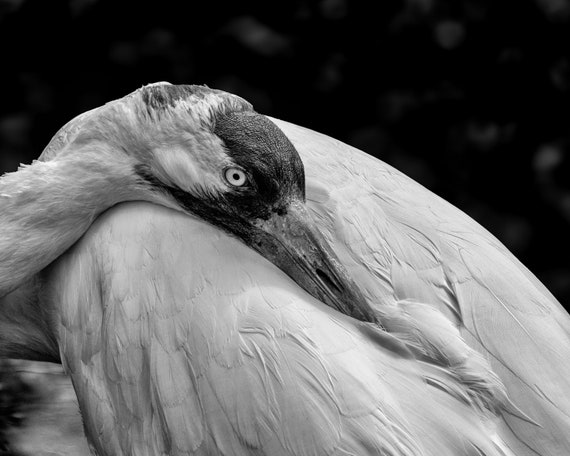This close-up black and white photograph features a bird, potentially a stork, swan, or flamingo, with its head tucked into its feathered body, creating a serene and introspective pose. The top third of the image is dominated by a stark black background which contrasts sharply with the bird's predominantly white feathers. From the cranium to just behind the eyes, the head is distinctively bald and smooth, covered in a dark black coloration, accentuating the small, pea-sized black pupil at the center of the eye. The bird's long neck is gracefully curved, with the beak turned and buried into the feathers on the back, giving a sense of restful repose. The texture of its feathers suggests a life adapted to water, reminiscent of species such as cranes or ducks. The composition highlights the elegance and tranquil nature of the bird against the minimalist, dark backdrop.